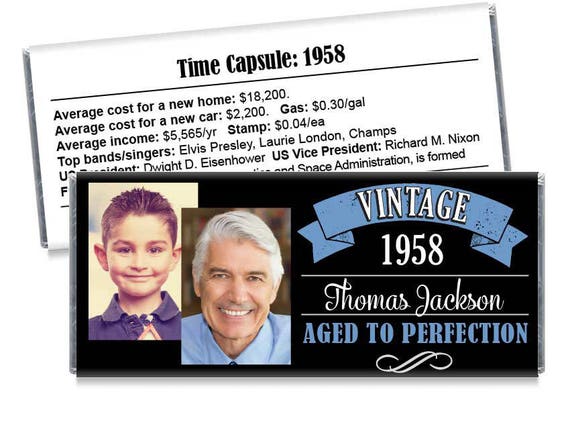This color photograph features two overlapping square cards, each providing a glimpse into the year 1958 and highlighting Thomas Jackson. The back card, set against a white background, presents "Time Capsule 1958" in bold black text, detailing notable statistics from that year: the average home cost was $18,200, a car was $2,200, gas cost 30 cents per gallon, the average annual income was $5,565, and a postage stamp was 4 cents. It lists popular musicians such as Elvis Presley, Lori London, and the Champs, and mentions U.S. President Dwight D. Eisenhower with Vice President Richard M. Nixon. Partially covering this card is a second one on a black background, featuring a photograph of a young boy and an older man, presumably Thomas Jackson at different ages. The card, adorned with a blue ribbon and white text, reads "Vintage 1958, Thomas Jackson, Aged to Perfection."